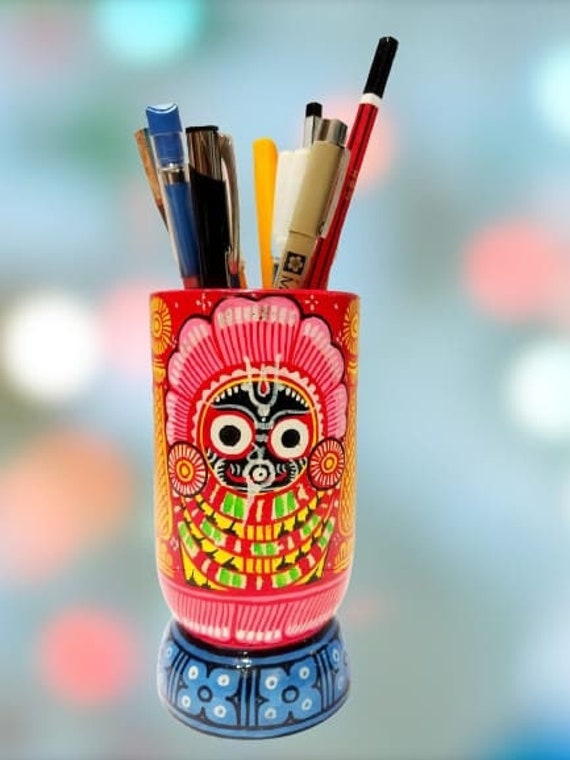The image depicts a vibrant and intricately designed pen and pencil holder. The tall, narrow container features a rich, cultural motif reminiscent of a tiki head or Aztec mask. The mask is adorned with a striking red headdress and detailed with red, black, white, and yellow colors. It also includes elements resembling feathers and vibrant necklaces in red and green hues. The base of the holder showcases an elegant blue floral pattern, transitioning into delicate pink stripes above. The container is filled with about eight assorted pens and pencils, contributing to the colorful display. The background is intentionally blurred, awash in soothing tones of blue, pink, light orange, and white, creating a soft, out-of-focus aesthetic that highlights the detailed artistry of the pen and pencil holder.